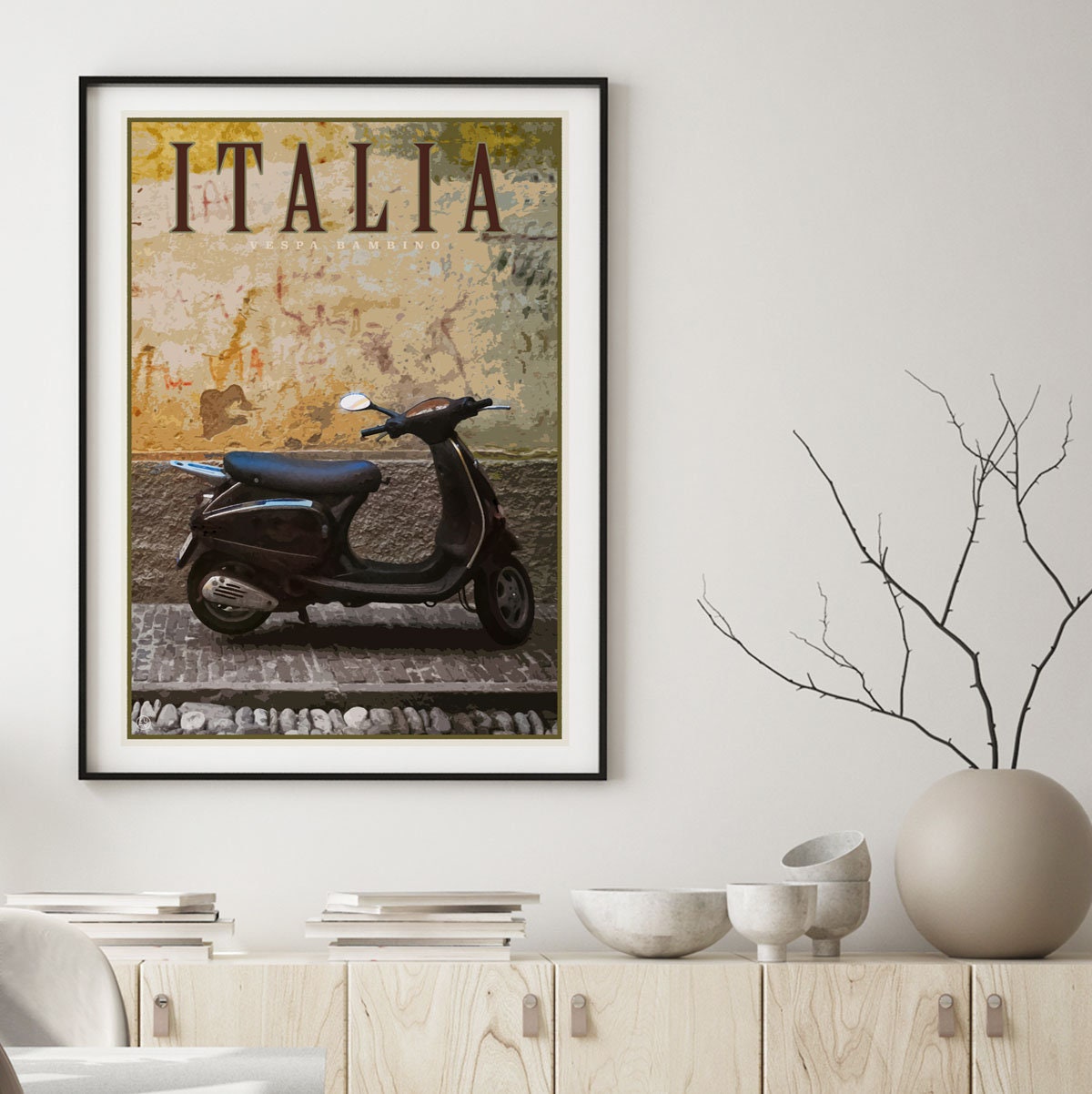This is a richly detailed image capturing a stylish interior scene. A light gray wall hosts a black-framed poster with a white mat. The poster prominently features the text "Italia" in bold black letters and "Vespa Bambino" in tan letters. Below the text is an evocative image of a black Vespa scooter positioned on gray cobblestones, set against a weathered, patina-rich backdrop with hues of yellow, beige, and green, evoking an ancient European ambiance.

Beneath the poster, a sleek credenza made of blonde, light-colored wood displays an arrangement of decor items. These include marble bowls, a spherical vase with bare branches, and a stack of nondescript white and beige books. To the left, the corners of a light gray chair and table are also visible. The overall palette of the room is cohesive, with light gray walls complementing the wooden and decorative elements, enhancing the elegance of the space.